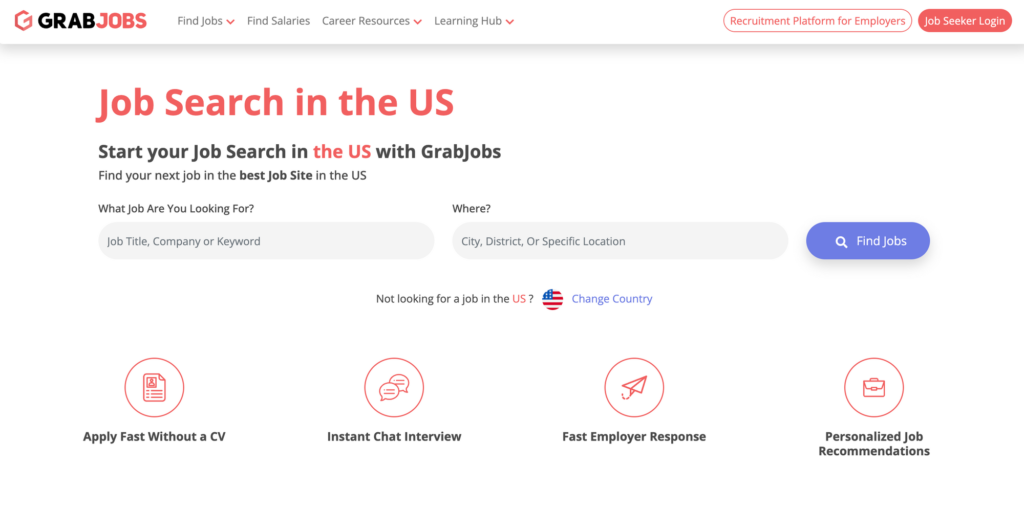The image appears to be a screenshot from the GrabJobs website, prominently featuring their branding and navigation sections. 

In the top-left corner, a red "G" logo is accompanied by the text "Grab" in black and "Jobs" in light red, signifying the GrabJobs website. Adjacent to this, four categories in gray are listed: "Find Jobs," "Find Salaries," "Career Resources," and "Learning Hub." To the right, in red, it reads "Recruitment Platform for Employers," followed by a "Job Seeker Login" button in white text on a red background. 

The main focal area of the website header displays "Job Search in the US" in large red letters. Directly underneath, in black, it states, "Start your job search in the US with GrabJobs," with "US" highlighted in red. Further down, it reads, "Find your next job in the best job site in the US."

Beneath this, there's a prompt in black text asking, "What are you looking for?" followed by a search bar with a gray background that says, "Job title, company, or keyword." To the right, a smaller black text asks, "Where?" with a search bar below it indicating "City, district, or specific location." Next to this search bar, a blue emblem displays "Find Jobs."

Below these search sections, the website offers additional options: "Not looking for a job in the US?" alongside a prompt to "Change Country." Underneath are several features enhanced by red emblems: "Apply Fast Without a CV," "Instant Chat Interview," "Fast Employer Response," and "Personalized Job Recommendations."